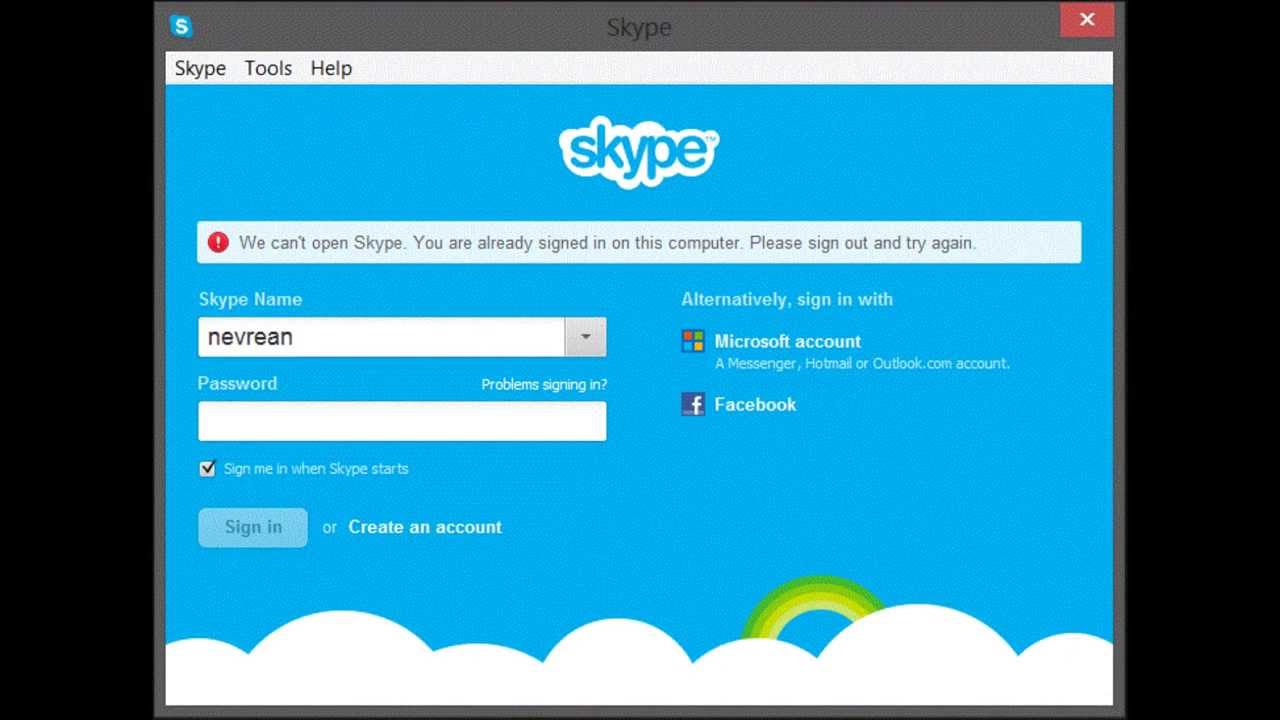This is a detailed screenshot of a Skype login window. The interface is characterized by a central section for inputting login credentials. The Skype name field is filled in with "neverine," but the password field remains empty. Additional login options are available on the right, allowing users to sign in with a Microsoft or Facebook account. 

The top portion of the window features the recognizable Skype logo set against a cloud-themed background, with the logo and text in blue hues. On the top-right corner, there's an "X" icon for closing the window, and on the top-left, navigation tabs for "Skype," "Tools," and "Help" can be seen.

At the bottom, a checkbox option labeled "Sign me in when Skype starts" is ticked, indicating the user wishes to stay signed in automatically. The background at the bottom includes whimsical cloud imagery with a green sun peeking through, adding a touch of visual flair to the interface.